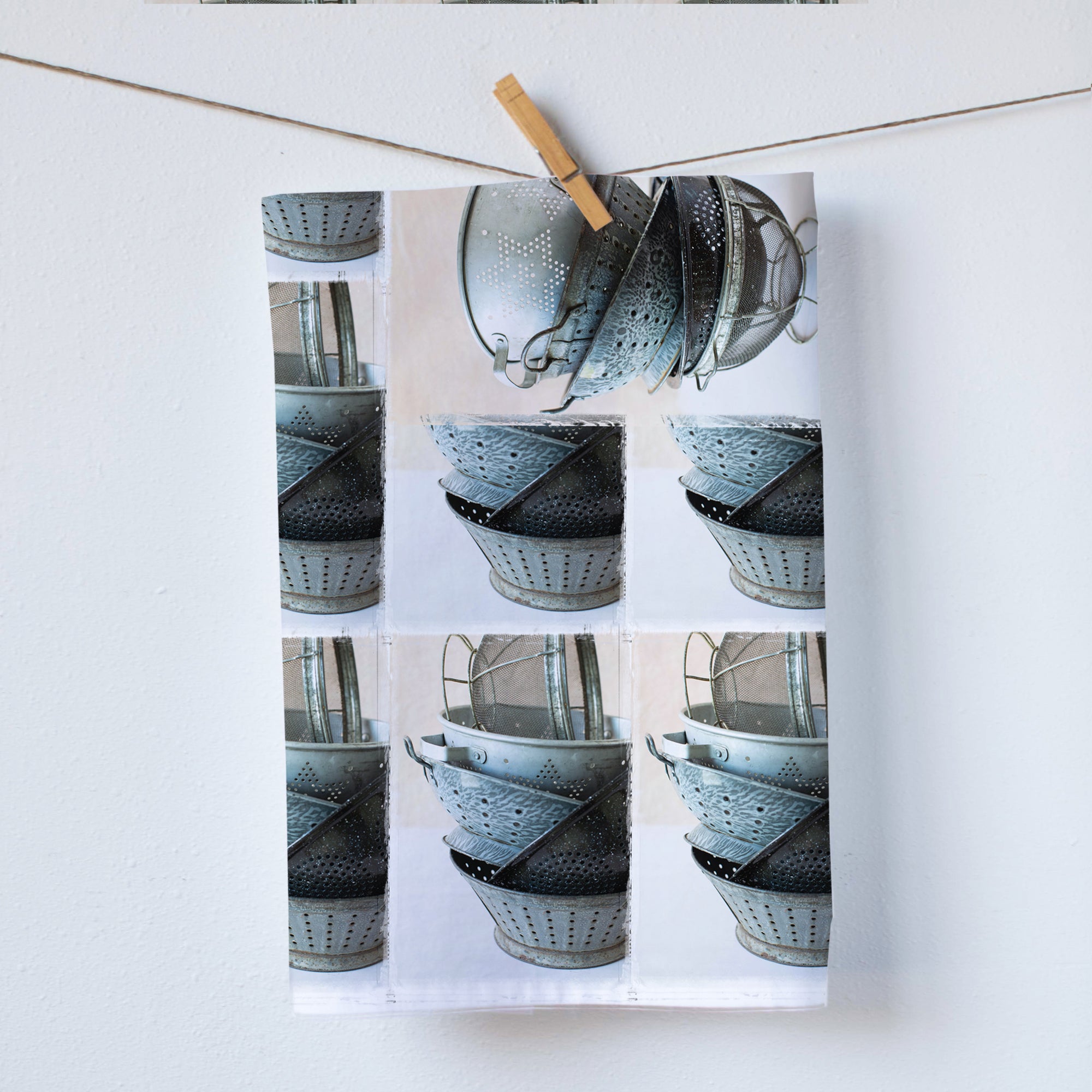This image captures a photograph clipped to a thin wire with a singular brown clothespin, set against a neutral-colored wall. The photograph itself showcases numerous kitchen utensils, prominently colanders, depicted in an organized yet somewhat haphazard display. The utensils, varying in copper and tin colors with some showing a bluish tint, are arranged in multiple rows across the image. The backdrop of the photograph is a subtle beige, helping the metallic hues of the colanders and other items to stand out. In total, there appear to be around eight panels within the photograph, each depicting different arrangements or segments of colanders and potentially other kitchen items, creating an intricate and detailed visual of everyday kitchenware.